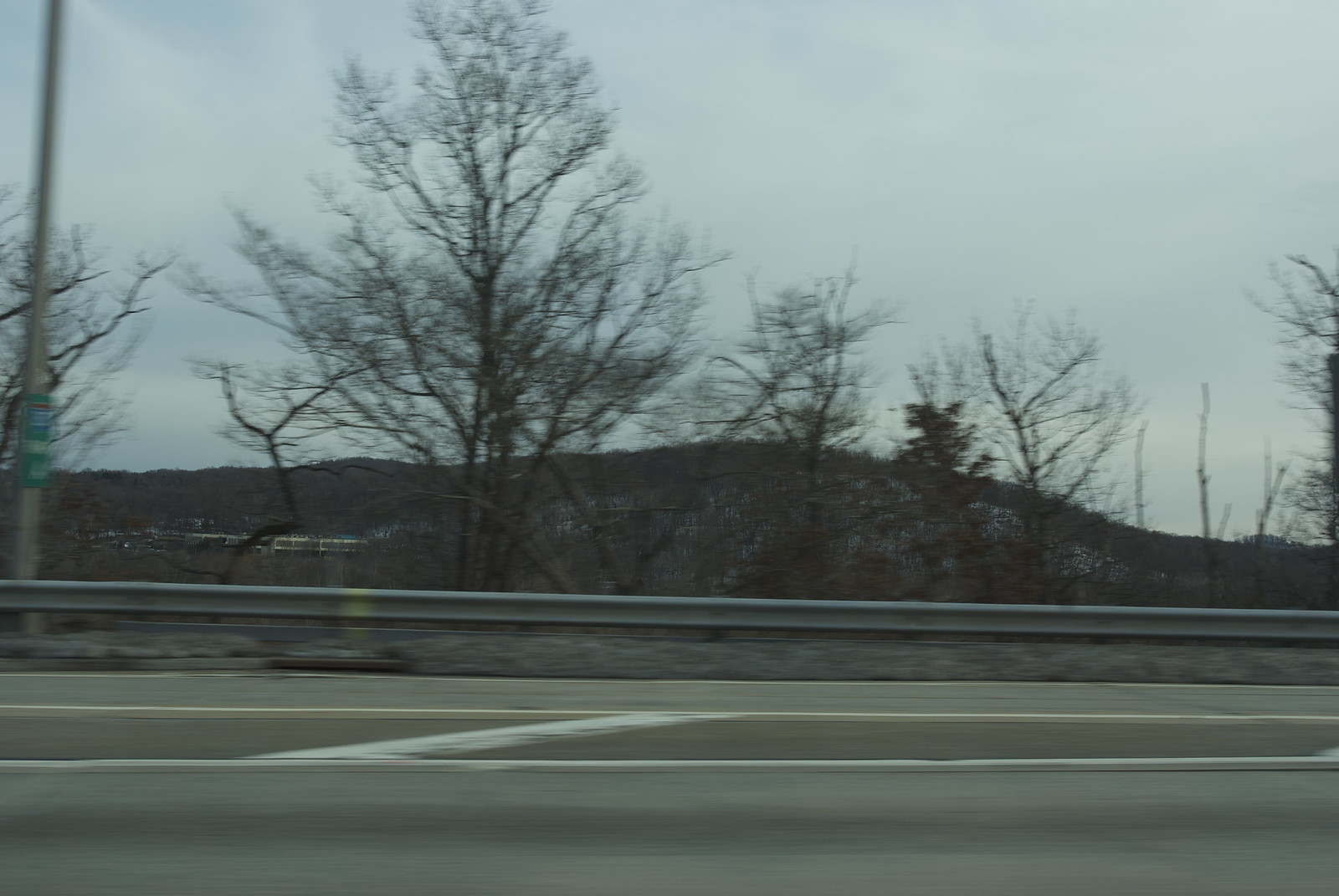This image, captured on a bleak, overcast day, depicts a dreary highway scene. The photograph features a view across a two-lane road with a dark median line marking the center. There are no vehicles on the road's concrete surface, creating a sense of emptiness. In the foreground, a strip of grass lies just before a metal guardrail that runs the length of the scene. Beyond the guardrail, numerous barren trees, devoid of leaves, suggest it is winter. Among these scraggly trees stands one notable pine tree with a sparse bit of greenery. The backdrop reveals low, rolling hills and a mountainous area, lending a sense of distance. On the left side of the image, there are some structures in the distance, situated against the hilly landscape under a heavy, whitish-gray sky. The photograph captures the stark and somber atmosphere of the setting.